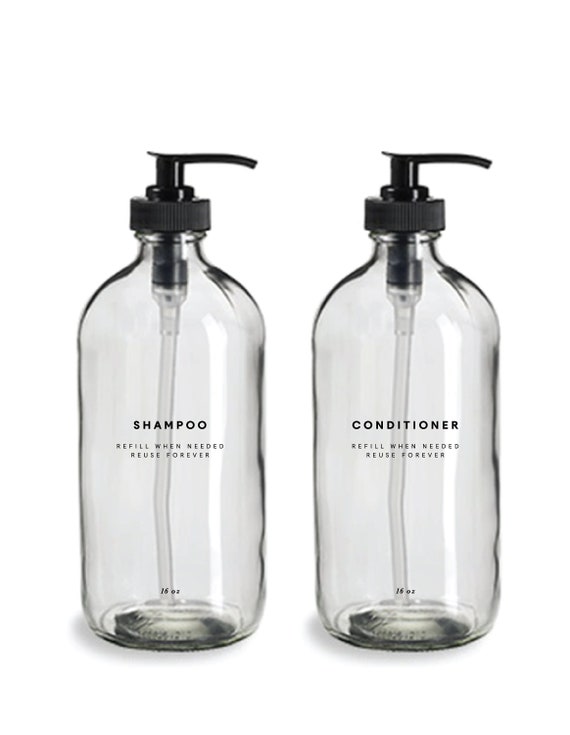The image depicts two clear, shiny bottles labeled "Shampoo" and "Conditioner" with black screw-on tops featuring pump dispensers. These reusable containers are designed for continuous refilling, as indicated by the text on both bottles: "refill when needed, reuse forever." The bottles share an identical design and appear to be made of hard plastic or glass. Each bottle is transparent, allowing visibility of the empty interiors and the pump tubes inside. Set against a white background, these sleek and eco-friendly bottles aim to reduce waste by promoting sustainable practices.